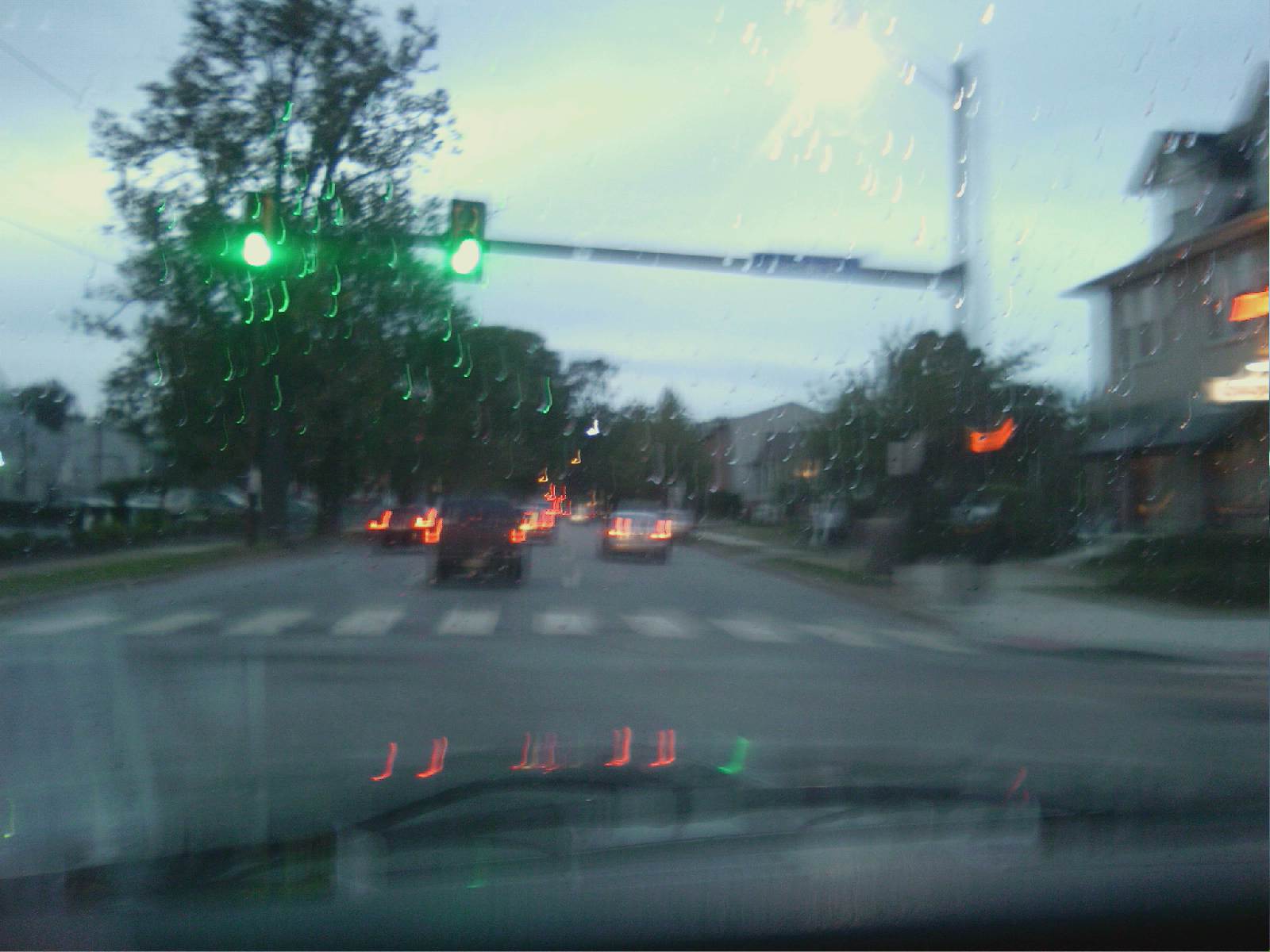In this slightly blurry photo, taken from the inside of a car, one can see a rainy day at a four-way intersection. The windshield wipers are in view, indicating it’s raining, with raindrops visible on the glass. The traffic light overhead displays green, signaling for the car to proceed, while red tail lights of vehicles are seen ahead, indicating other cars have stopped across the intersection. No pedestrians are seen on the white crosswalk lines. On the left side of the road, a sidewalk bordered by green grass lines the street with a few blurred buildings or vehicles in the background. To the right, there are additional buildings which include a shop or restaurant with its lights on, and there are trees and more grassy areas along the sidewalk. The scene is cast in a hazy light, possibly due to the rain and motion blur, giving an impression of a typical overcast day on a city road.